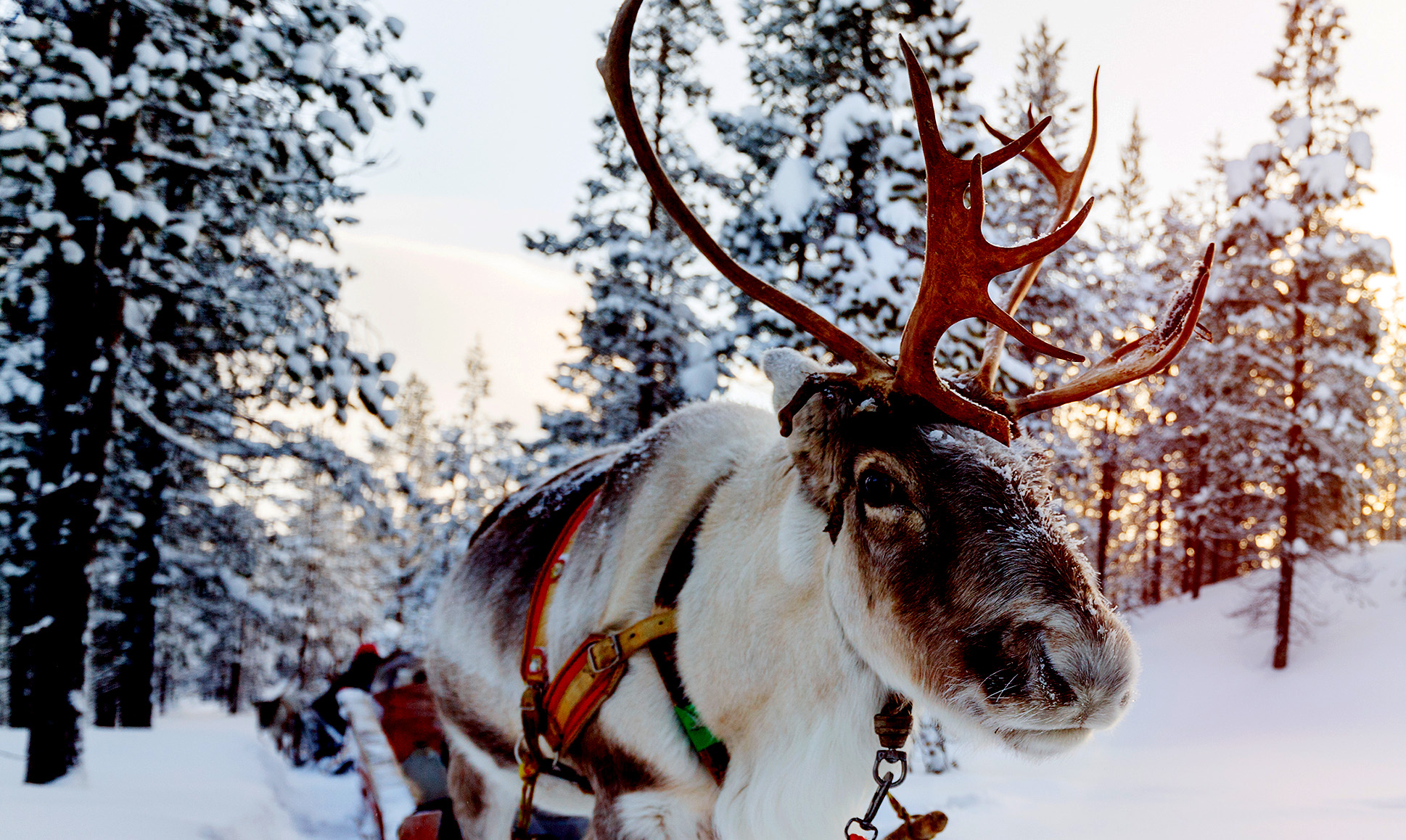This striking photograph captures a reindeer standing in a snowy, winter landscape. The reindeer, with a brown and white mottled coat, gazes directly at the camera, revealing only its right eye. Its large antlers appear light brown, likely due to the sunlight reflecting in the top right corner of the image. The reindeer is adorned with a vibrant harness featuring black, red, and gold leather strips with silver embellishments, and bells hang from its neck. Snow-covered pine trees and a bright, pale blue sky with scattered clouds form the blurred backdrop. The ground around the reindeer is blanketed in snow, with footprints visible in the bottom left corner. Behind the reindeer, a sleigh can be seen, though it is slightly blurred, and a shadowy figure is discernible, suggesting that the reindeer is part of a winter sleigh ride scene. But what truly stands out is how the reindeer, with a touch of snow on its face and body, leads this picturesque, sunlit winter tableau.